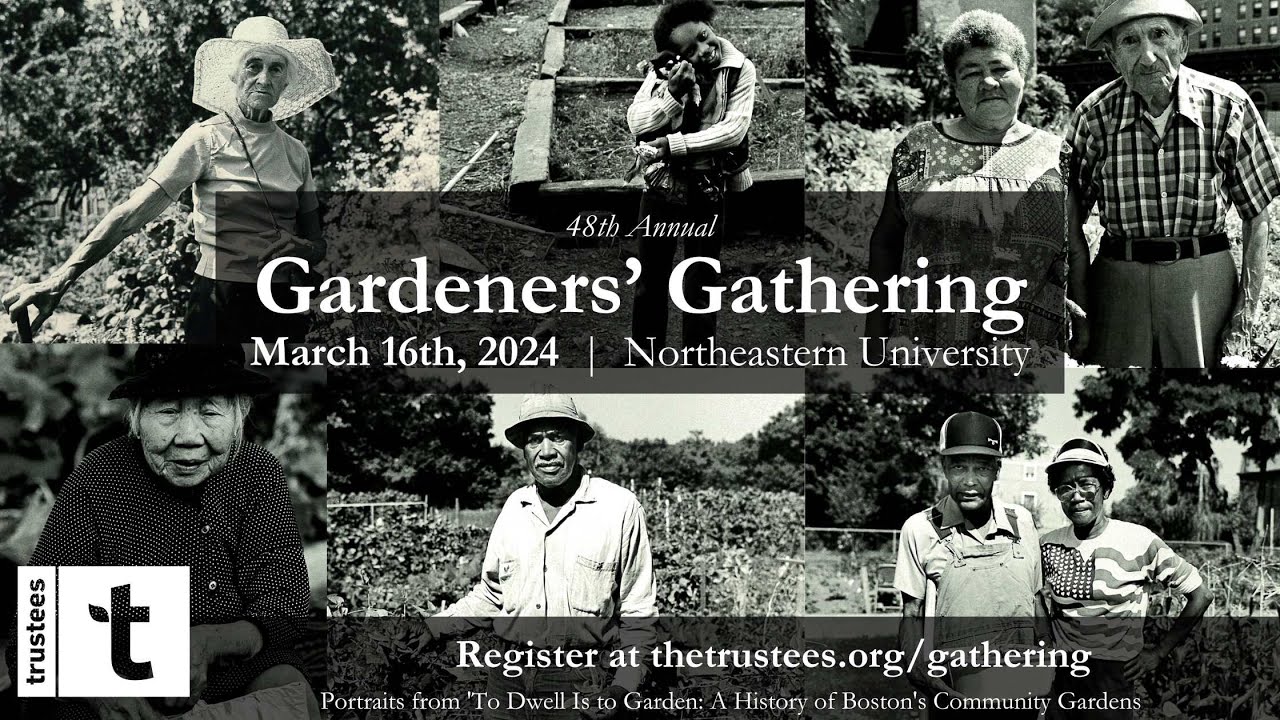The black-and-white advertisement for the 48th Annual Gardeners' Gathering, set for March 16th, 2024, at Northeastern University, is a collage of six distinct portraits showcasing diverse individuals in garden-like settings. At the center of this horizontal rectangle image, bold white text announces the event details. Below this, a banner provides further information, urging viewers to register at "thetrustees.org/gathering" and mentioning that the event will feature "portraits from To Dwell is to Garden, a history of Boston's community gardens." The bottom-left corner displays the logo of The Trustees, featuring a stylized 'T' with a leaf. From left to right, the collage includes: a person in a white sun hat and light t-shirt, a Black woman holding and hugging an animal, a white couple, an elderly Asian woman in dark attire, a tan-skinned man in a long-sleeved white shirt and hat, and a Black couple, all of whom are likely gardeners or enthusiasts.